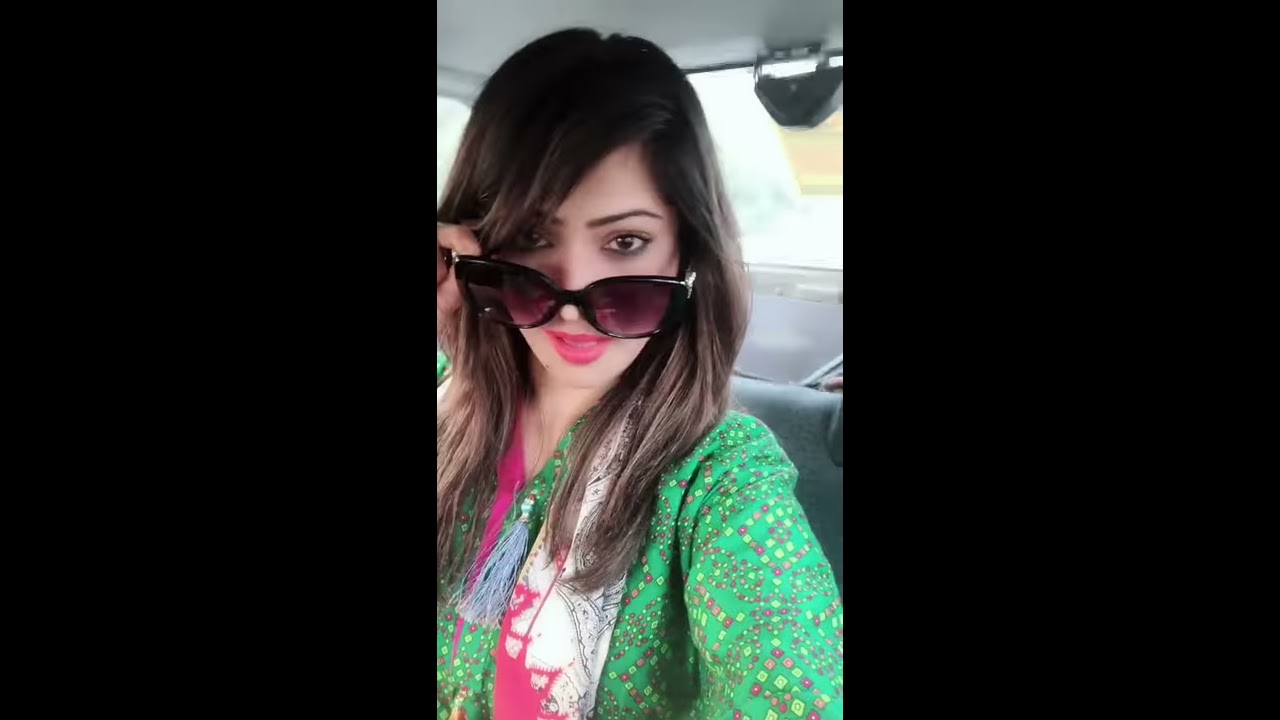The image is a detailed selfie of a woman inside a vehicle, likely a taxi or ride-share. She holds her phone extended with her left arm, capturing her face and upper torso. She is dressed modestly in a long-sleeve green top adorned with intricate pink and green triangle designs. Adding some flair, she sports a white and pink striped scarf with a blue tassel. Her dark brown hair is parted from left to right, and her thin, tweezed eyebrows frame her brown eyes, highlighted by minimal makeup. Her lips are colored with thick light pink lipstick. She wears dark purple-lensed sunglasses, which she has pulled down to the tip of her nose to expose her eyes seductively to the camera. The vehicle's interior features dark gray fabric seats with a lighter gray roof, suggesting a typical car setting. The photo's aspect ratio suggests it might be a screenshot from a live stream, and the image is well-lit by natural daytime light, enhancing its clarity and brightness.